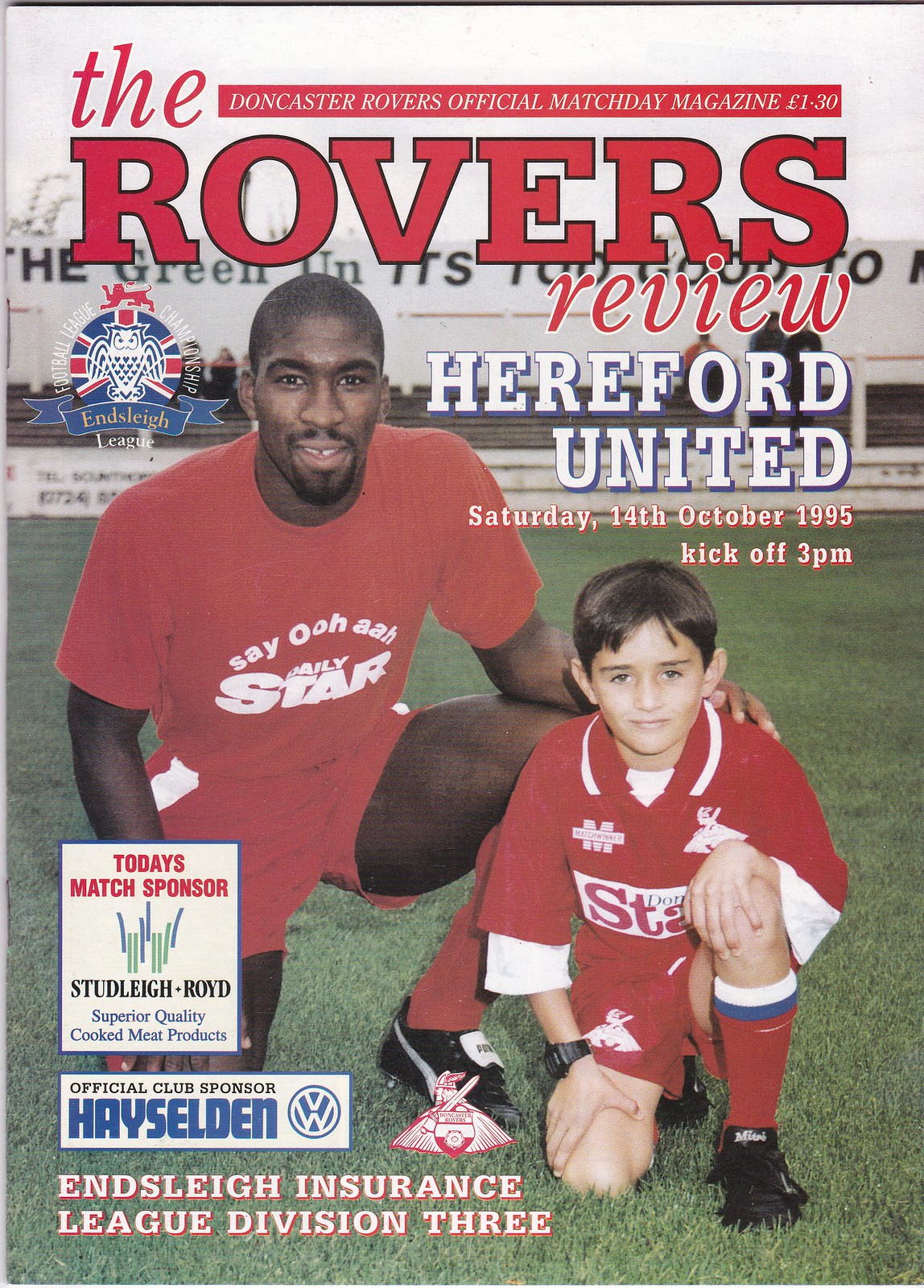This magazine cover, titled "The Rover's Review," is the official match day publication for Doncaster Rovers, featuring the match against Hereford United on Saturday, October 14, 1995, with a kickoff at 3 p.m. At the very top, it is labeled as the Doncaster Rovers Official Match Day Magazine, priced at £1-30.

Prominently displayed on the cover are an athlete and a young boy, both dressed in red uniforms. The athlete, a black man with a short haircut, mustache, and goatee, is down on one knee with the other knee raised. He wears a red shirt with the words "Say Ooh Ah Daily Star" across it, red shorts, red socks, and black cleats. The athlete has a gap-toothed smile and his arm affectionately rests on the shoulder of the young boy beside him.

The young boy, a white child with brown hair parted in the center, mirrors the man's pose with one knee down. He sports a red shirt displaying the letters "S.T.A." and an emblem that resembles a deer, along with red shorts and black shoes. Both appear happy, sitting on a grassy field with bleachers and spectators in the background. A white wall behind them features the text "H.E. Green" and some foreign language lettering.

At the bottom left of the cover, there are advertisements: "Today's Match Sponsor, Studley Boyd, Superior Quality Cooked Meat Products," followed by "Official Club Sponsor, Iceland" with a Volkswagen logo, and "Ensley Insurance, League Division III."